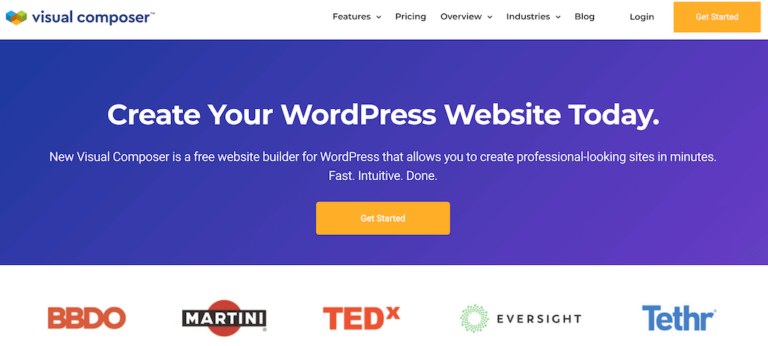The top left of the website features a logo with "Visual Composer" accompanied by a trademark symbol. The logo consists of three interlocking blocks forming a heart shape: a blue block at the top left, an orange block at the bottom, and a green block at the top right. The "Visual Composer" text appears in bold purple letters.

To the right of the logo is a navigation menu with options: Features, Pricing, Overview, Industries, Blog, and Login. The menu items "Features," "Overview," and "Industries" have a drop-down arrow next to them. An orange rectangular button with white lettering reads "Get Started."

A large dark purple filled rectangle spans the top of the page, bearing the message: "Create your WordPress website today." in bold white letters. Below this, in smaller, non-bold white text, it reads: "New Visual Composer is a free website builder for WordPress that allows you to create professional-looking sites in minutes. Fast. Intuitive. Done." An orange-yellow rectangular box underneath this text says "Get Started" in white.

At the bottom left, the website features several logos: the letters "BB" in bold, capitalized, red rounded font; a red circle with a black rectangle and "martini" in white, capital letters; the TEDx logo; the "Eversight" logo with spaced-out letters; and a lime green floral design next to the blue bold text "Teeth".